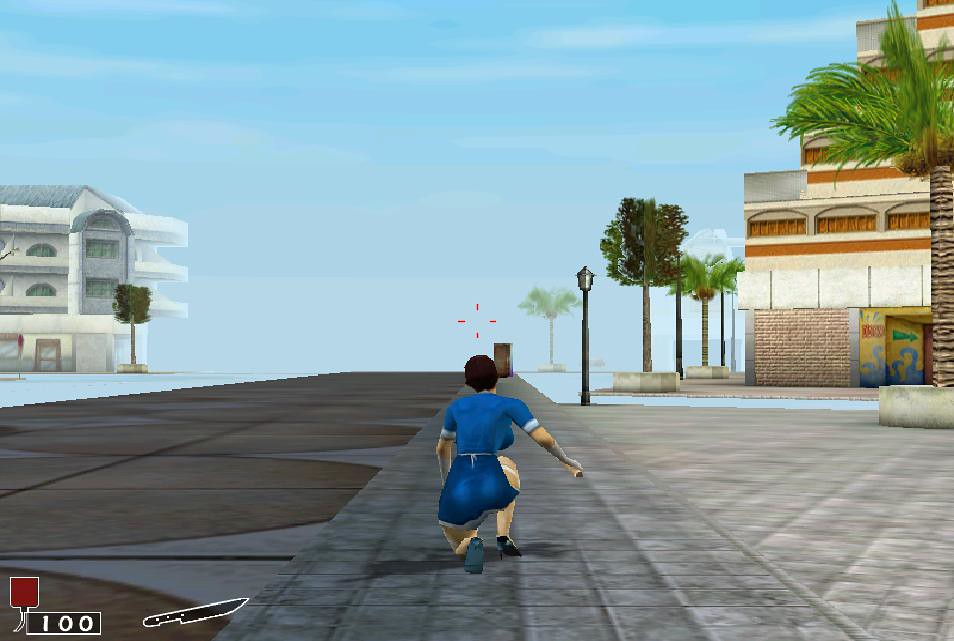This screenshot is from a digital game, showcasing a scene centered around the player character, who appears to be a white or light-skinned female. She is positioned slightly towards the bottom center of the screen and is dressed in a short blue outfit adorned with white trim on the ends of the dress and sleeves. The character, seen from behind, has a red crosshair above her head made up of four dashes, signifying potential targeting or focus.

The setting seems to be a commercial area with a cement brick pathway beneath the character. On the left side, the pavement has a different pattern, while on the right it transitions into a diamond pattern. Palm trees in cement planters enhance the urban aesthetic. To the right, there is a partially visible building made of brick, painted red, beige, and white with a green and yellow entrance sign just visible on the image’s edge.

On the left, another building resembling an apartment complex or residential area is partly loaded, with some missing ground textures, giving an impression of cement floating on water against a blue sky backdrop. The sky is bright, featuring wispy clouds, indicating a daylight scene.

Additionally, the game’s user interface (UI) is visible at the bottom left corner, featuring sparse elements: a black rectangle with a white outline displaying the number "100," a red symbol resembling a square balloon, and a black silhouette of a kitchen knife outlined in white with three dots beside it.